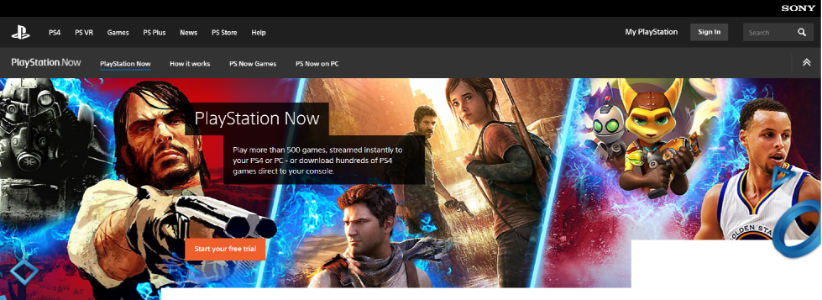A highly detailed screenshot captured from a web browser shows the PlayStation Store interface. Prominently featuring the PlayStation logo on the top left corner, the logo creatively merges the letters "P" and "S" with the "P" standing upright and the "S" lying horizontally. Adjacent to the logo, a horizontal navigation bar houses several category buttons, including "PS4," "PSVR," "Games," "PS Plus," "News," "PlayStation Store," and "Help."

Dominating the center of the screenshot is an expansive banner adorned with vibrant images of various video game characters. Among these characters, an older man accompanies a younger woman, signaling an emotional storyline, while another segment of the banner showcases a professional basketball player in action. Additionally, a character brandishes a formidable double-barrel gun, hinting at intense gameplay scenarios.

Positioned in the top right corner are the Sony logo and a small, functional search bar for easy navigation. There is also a conspicuous 'Sign In' button, likely to access personal accounts. The website's overall aesthetic is sleek and modern, utilizing a dark theme with a blend of black and dark gray for the background, which contrasts elegantly with the colorful banner and navigational elements.